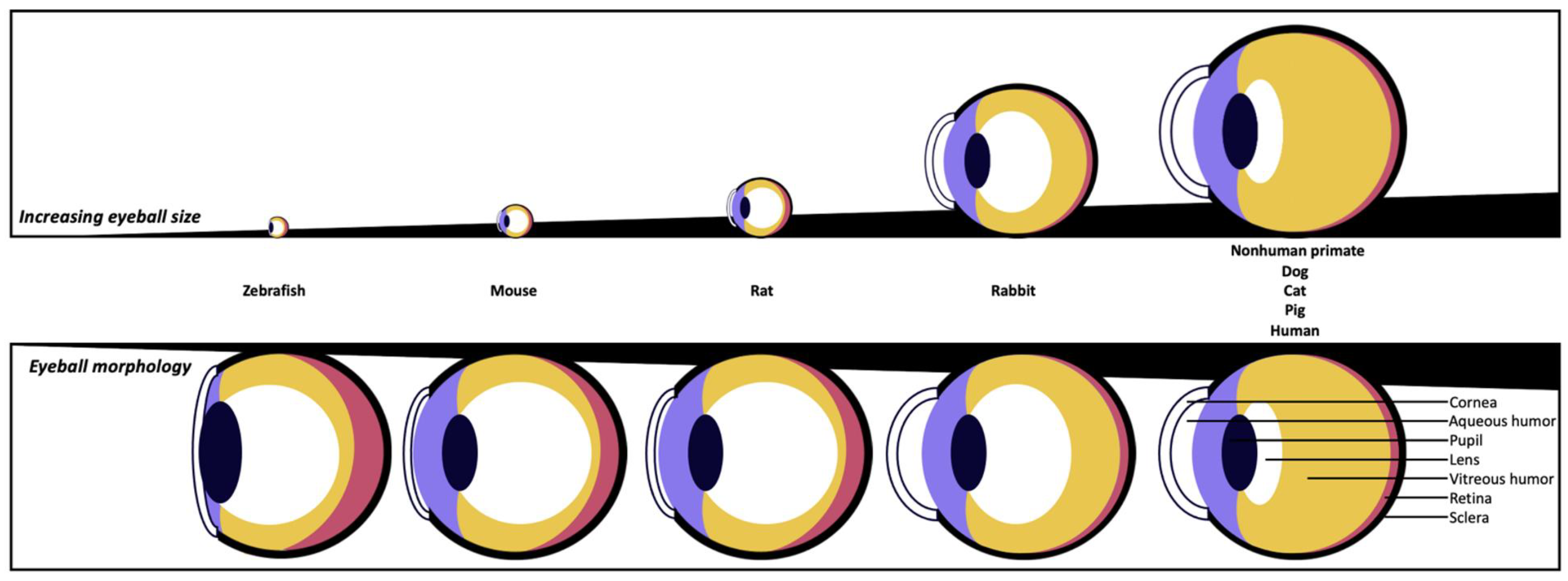The image presents a graphical depiction of increasing eyeball size across various animals, arranged from left to right starting with zebrafish and progressively moving through mouse, rat, rabbit, and continuing to non-human primates such as dogs, cats, and pigs, culminating with humans who have the largest eyes. The top row features eyeball representations that grow in size sequentially. The accompanying bottom row illustrates the morphology of the eyeball, detailing its anatomical components—cornea, aqueous humor, pupil, lens, vitreous humor, retina, and sclera—which become more distinct and circular as the eyeball size increases. Each detailed segment underscores the comparative anatomy and evolution of the eye across species, depicted in a visually informative manner.